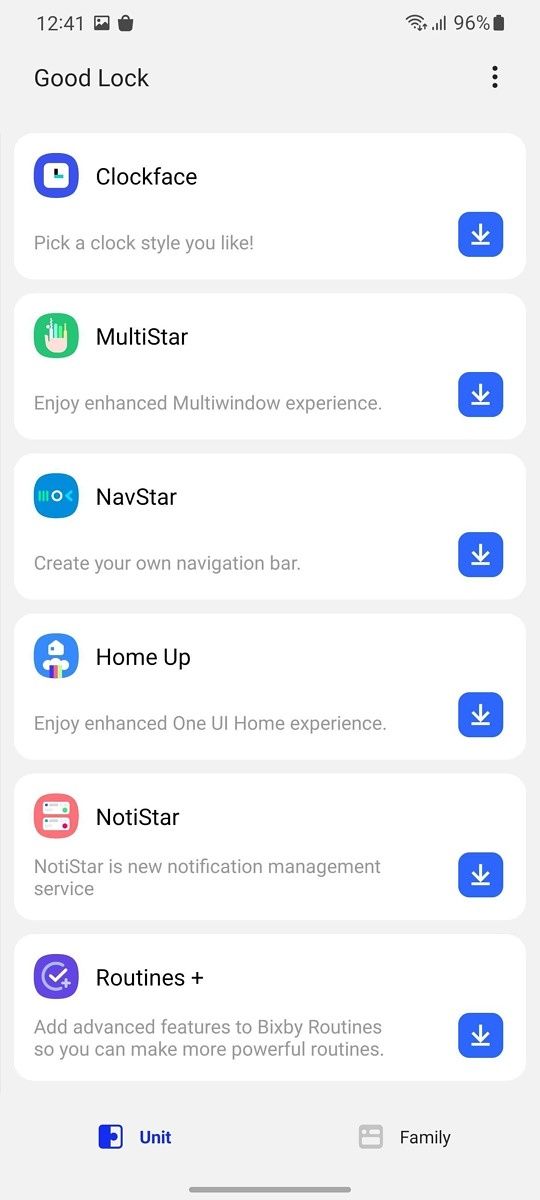### Detailed Caption for the Image:

"This image showcases an app presumably designed for Samsung phones, aimed at enhancing and customizing the user interface, particularly the lock screen and home screen. The top section features options for selecting different clock styles, allowing users to personalize their clock face. Below this section is an option labeled "Multi-Star," which promises an enhanced multi-window experience, along with a prompt to download the feature.

Further down is the "NavStar" option, encouraging users to create their own custom navigation bar, followed by a download button. The "Home Up" feature aims to provide an enriched user interface home experience, also available for download. Another feature named "NotiStar" offers an advanced notification management service, adding another layer of customization for notifications, again with a download prompt.

The final section highlights "Routines+" which adds advanced features to Samsung's Bixby assistant, enabling users to craft more powerful and personalized routines. The bottom of the image contains the terms "Unit" and "Family," suggesting categories or feature sets within the app. This image appears to be a promotional interface or menu for a Bixby customization tool designed to enhance the functionality and personalization of a Samsung device."